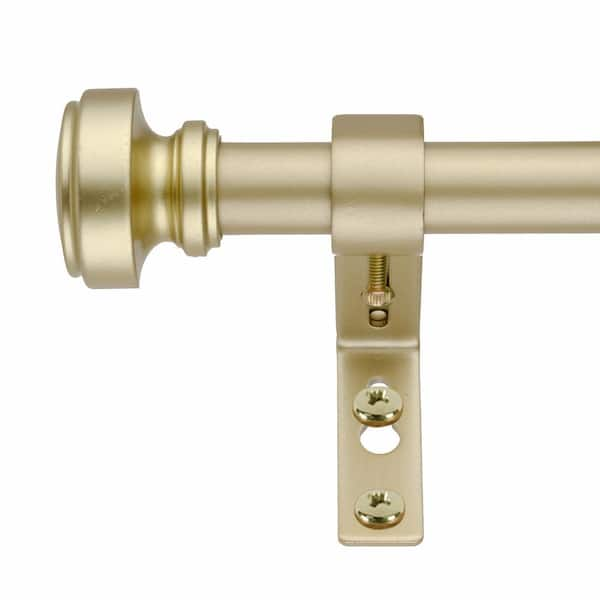This image captures a detailed, close-up view of the left end of a gold curtain rod, photographed from an upward angle as if standing directly beneath it. The rod itself is made of metallic gold, with a matte finish, while the finial at the end is a shiny, brighter yellow gold. The finial is intricately designed with a disc on the outermost edge, followed by a larger, wider disc, and then a series of three smaller discs tapering down before attaching to the rod. 

The bracket supporting the rod is of the arm style, also finished in matte gold. It affixes to the wall with two screws. The bracket has a flat metal arm curving downward, creating a cradle for the rod. There is a screw going up into the bottom of the bracket to secure its position on the rod. The bottom of the bracket features two holes: one with a screw already in place and another keyhole-shaped for adjusting the bracket's position on the wall. The matte gold finish of the rod and bracket contrasts with the bright, reflective gold screws and the vibrant finial, making this a visually detailed and decorative piece.